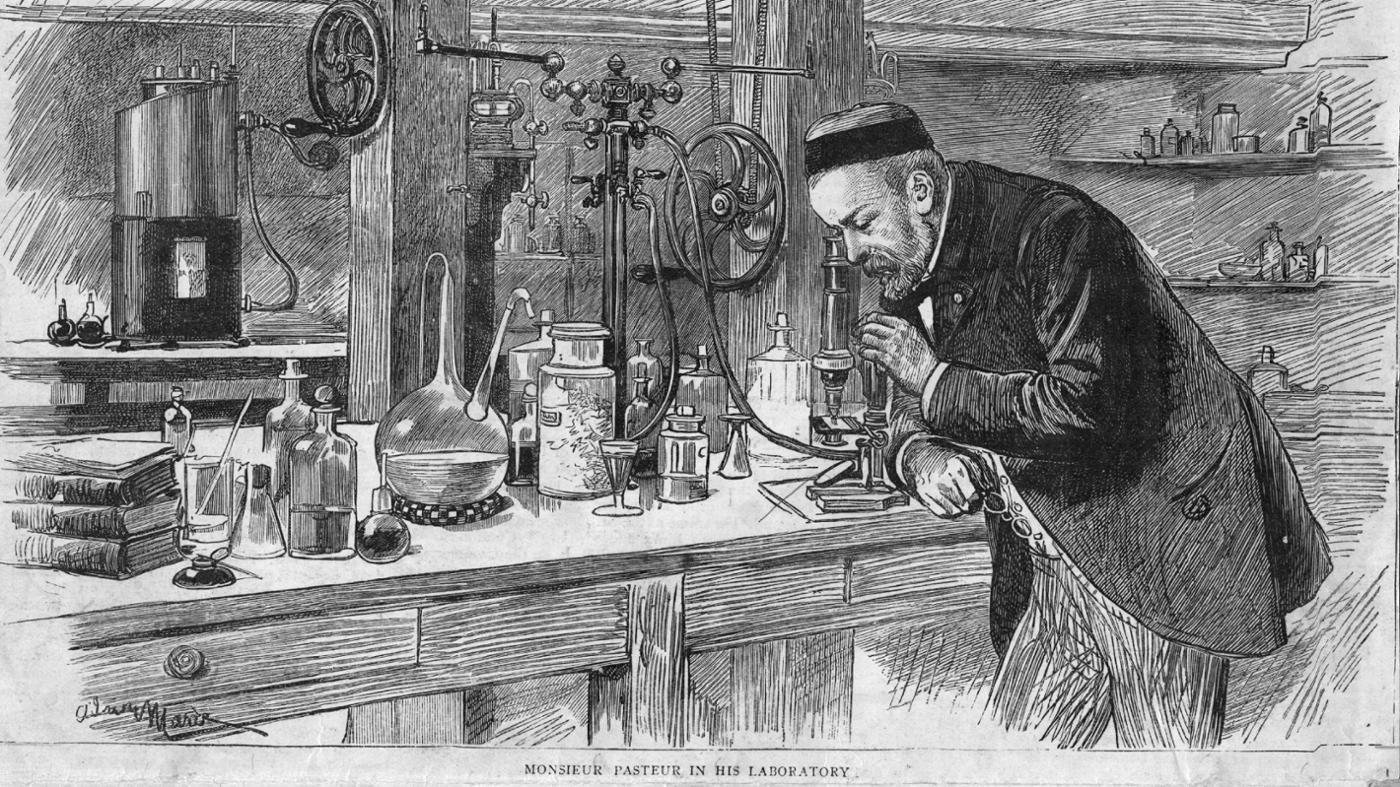This is a detailed, hand-drawn, horizontally aligned rectangular sketch depicting a man identified by the text at the bottom as "Monsieur Pasteur in his laboratory." The scene is set in the late 1800s or early 1900s and is rendered in grayscale with heavy shading techniques using pencil. Monsieur Pasteur, assumed to be French, is shown wearing a black coat and gray trousers, along with a black headband, which gives an impression of intense concentration. He is engaged in a chemical experiment, kneeling and looking through an early microscope that is part of a larger contraption.

The laboratory setting is meticulously detailed. The man is on the right side of the drawing, and a wooden counter with drawers featuring small knobs is visible. On the top of this counter, numerous flasks, beakers, and other glass containers, some filled with liquids, are spread out. A distinctive large glass flask with a narrow top is about half full. Additional scientific instruments, pill bottles, and books are scattered across the workspace. In the background, cylindrical equipment with hoses and wheels attached to wooden columns is also sketched in. Various shading techniques illustrate different textures and depths, with horizontal lines shading the drawers and vertical lines under the cabinets, while the walls combine diagonal and horizontal lines. The overall scene captures the essence of a historical laboratory bustling with scientific activity.